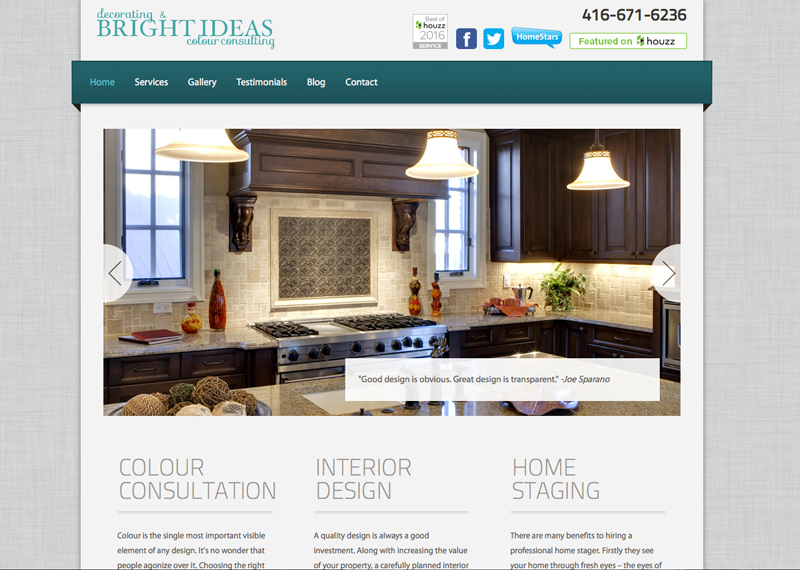**Detailed Caption for the Image:**

The image depicts the home page of a company called "Decorating and Bright Ideas Color Consulting." At the top of the page, the company's logo, "Bright Ideas" in light green, is positioned on the top left. Their contact number, 416-671-2636, is displayed on the upper right-hand side. They proudly showcase a "Best House Award 2016" badge near the logo. Links to Facebook, Twitter, and a Homestars feature are also visible on the page. The website options, which include Home, Services, Gallery, Testimonials, Blog, Ad, and Contact, are arranged in a dark green navigation bar across the top.

The current view is of the home page, which features an elegant kitchen. The kitchen has warm, brown cabinets, a gas top stove, marble countertops, and is decorated with plants and pepper shakers. At the center of the home page, a white box displays a quote: “Good design is obvious. Great design is transparent.” attributed to Joe Soprano.

Further down are three large menu options highlighting their main services: color consultation, interior design, and home staging. However, the text snippets cut off, leaving intriguing phrases like "Colors are the single most important viable element of the design...," "A carefully planned interior...," and "Firstly, they're home through the eyes of..." incomplete.

Overall, the page effectively introduces visitors to the company's color consulting services with a professional and visually appealing design.